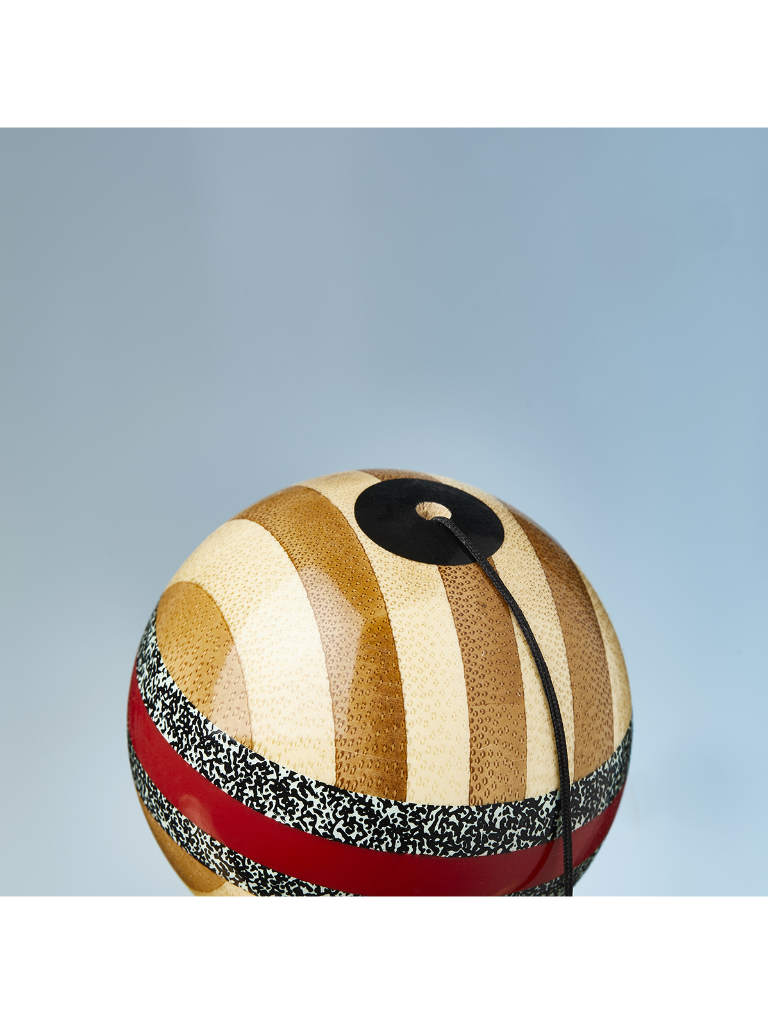The image features a detailed Christmas ornament, depicted as a spherical ball, with its bottom edge cropped by the photo border. The background is a gradient of dull blue transitioning into bluish gray toward the top. Vertically, the ornament is adorned with alternating gold and light white-yellow stripes that radiate from its edge. Horizontally, a central band composed of black and white dotted stripes, resembling a composition notebook pattern, spans the ornament, intersected by a solid red stripe. At the very top, there is a small black circle with an open center, from which a black string extends downward, crossing the front right side of the ornament and hanging off the edge of the image. The ornament, textured with tactile dots and markings, presents a vibrant contrast against the soft, muted background.